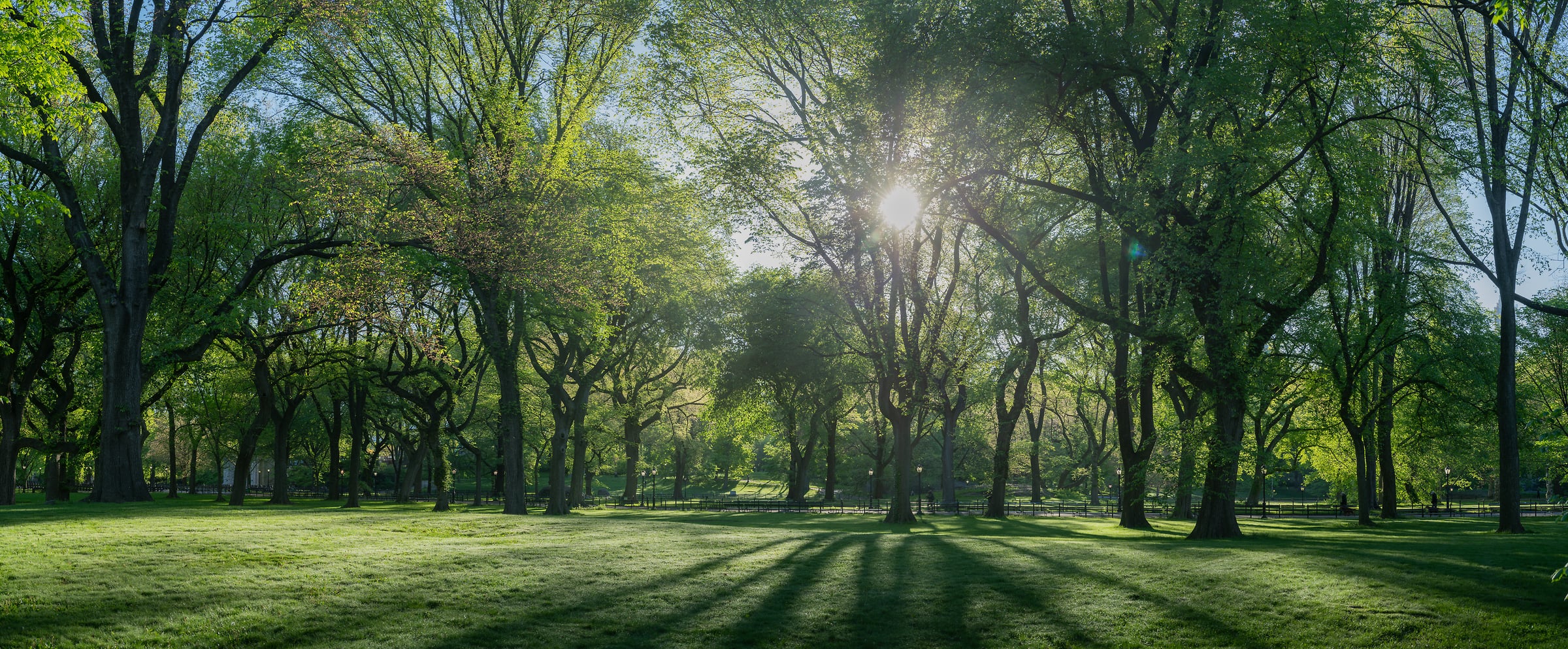The image captures a serene, sunlit scene in a well-maintained park, possibly Central Park in New York City. The foreground showcases a stretch of sun-kissed grass that is lush but slightly shaggy, enhancing the natural, park-like atmosphere. Multiple trees with vibrant green leaves and sturdy, darker limbs spread across the image, creating a dense yet welcoming canopy. The sun, positioned almost centrally, peeks through the middle tree, casting dramatic, long shadows that stretch towards the viewer, accentuating the tranquil setting. In the background, subtle details reveal park benches, streetlights, and a pathway where a solitary figure appears to be walking, all hinting at a quiet moment in late spring or early summer. The overall scene exudes an overwhelming green hue, underscoring the vitality and freshness of the park during this season.